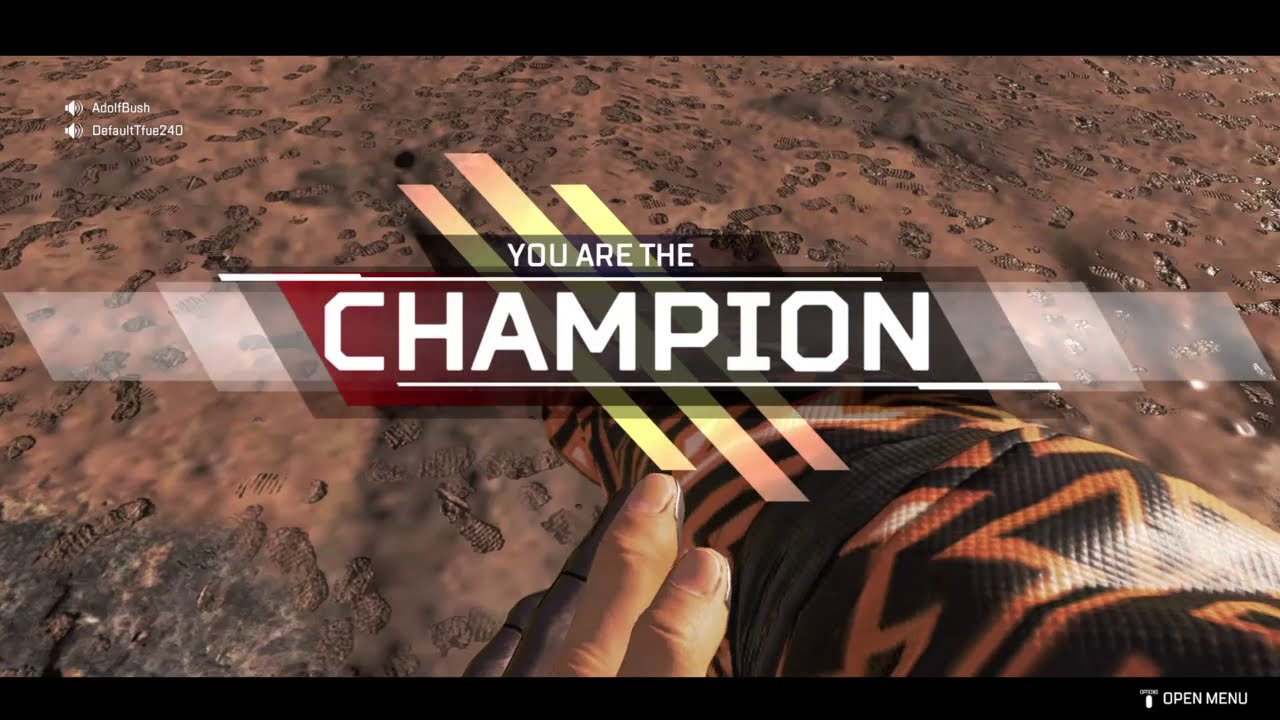This detailed descriptive caption integrates and highlights the shared elements from each voice caption:

This image captures a victorious moment from the video game Apex Legends, showcasing the winning screen. At the center, the prominent white text reads "You Are The Champion," with "You Are The" in a smaller font compared to "Champion." The text is set against a background featuring a pattern of orange with black and white triangles, reminiscent of snake skin, and is segmented by three diagonal stripes ascending from the bottom right to the upper left. In the upper left corner, smaller text displays a username including "Bush" and "default to 40." Additionally, a speaker icon is located nearby this text. The bottom right part of the screen features the option "Open Menu." The backdrop of the image is a dry, cracked dirt ground devoid of vegetation, adding to the game's intense atmosphere. A player's hand, adorned in a black and orange patterned sleeve, is lightly touching another hand, which is clearly visible to the viewer, enhancing the immersive first-person perspective of the game.